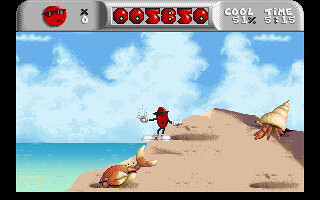The image appears to be a screenshot from a relatively primitive video game. Dominating the center is a character, depicted as a small red disc wearing sunglasses and sporting a black mouth. This character has thin, black stick-like arms and legs, culminating in large white hands and shoes. The scene is set on a large sandy hill at the beach, with turquoise ocean water visible to the right and a vibrant blue sky adorned with white, rounded clouds in the background. The foreground features two sea creatures: one appears to be a hermit crab with an extended claw, while the other resembles a crab partially emerging from the sand. At the top of the screen, there's a gray strip displaying a smaller version of the red disc character, along with game stats including a silver coin, an "X", and numbers like 005850, 51% cool, and a timer showing 515.